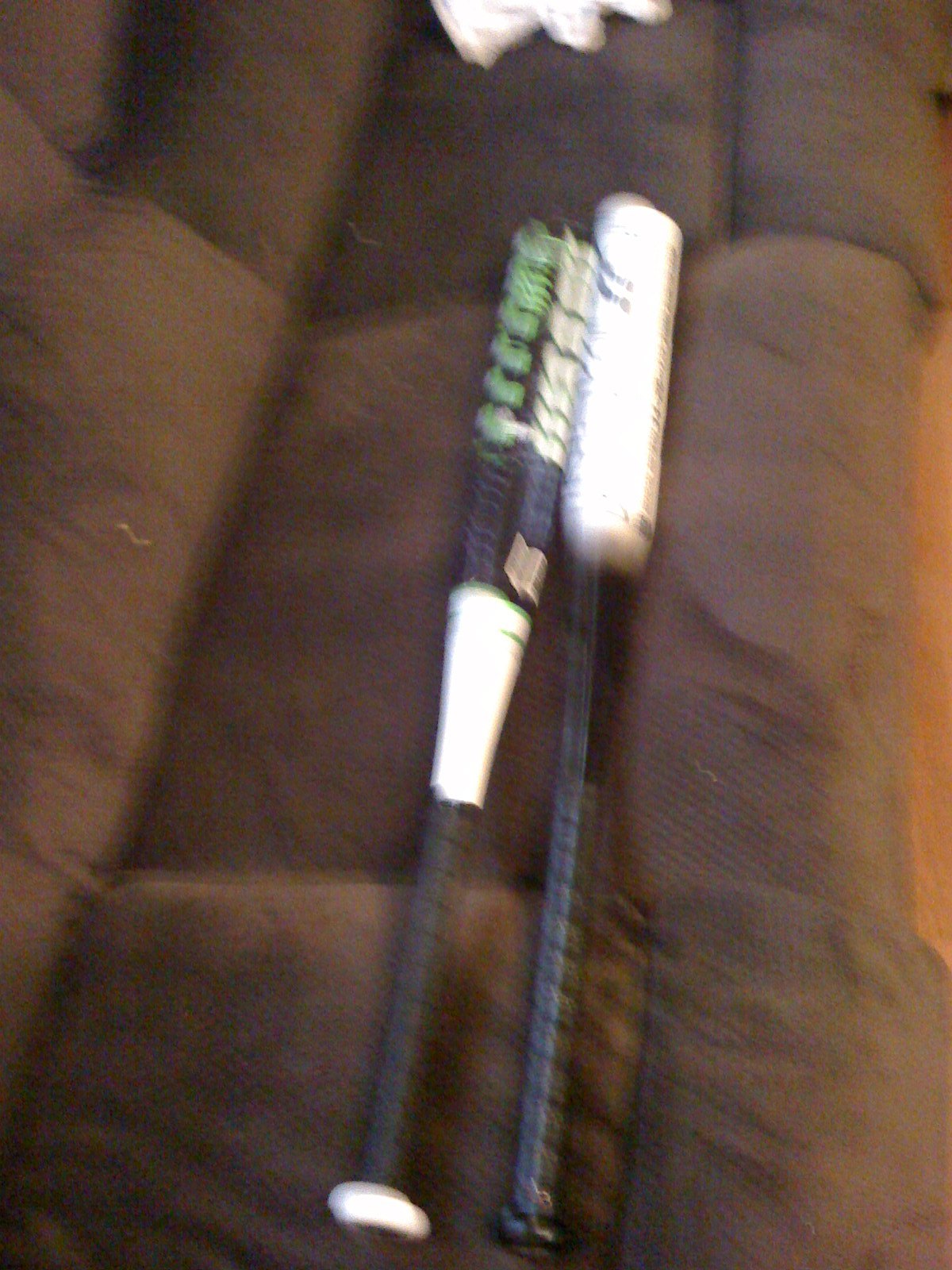The image, though quite blurry, depicts a scene indoors featuring a brown suede or velour sofa, possibly of the reclining variety, viewed from a slightly elevated side angle. On the sofa, there's a piece of white material at the top middle, possibly a glove or cloth of some kind. Prominently laid out on the main part of the sofa are two bats. The bat on the left features a detailed pattern with sections of black, white, and green, including black tape around the handle. The second bat, on the right, appears mostly black with a white top section. Despite the unclear image quality, the bats exhibit attributes more associated with cricket bats than baseball bats, such as their squarer top portion.